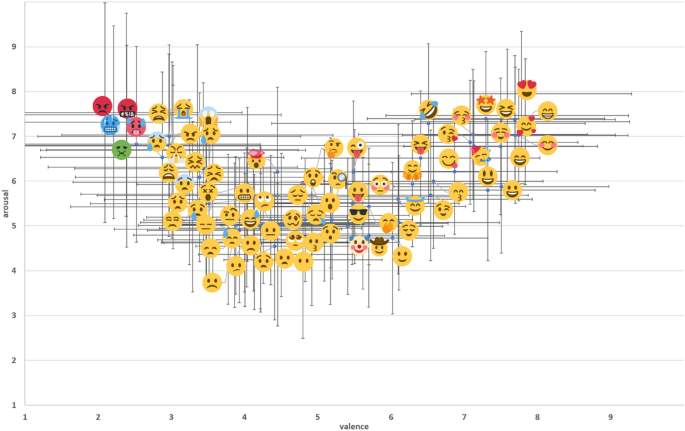This image depicts a graph with an x-axis labeled "Valence" and a y-axis labeled "Arousal." The scale on both axes ranges from 1 to 9. The graph, which uses a white background, is populated with various emojis, each representing different emotional states. 

Horizontal and vertical gray lines intersect through the emojis, clearly positioning them according to their arousal and valence values.

From left to right, the emojis are:

- Two red angry emojis, indicating high arousal and negative valence.
- A blue emoji with a grim expression showing all its teeth, also in the negative valence region with moderate arousal.
- A pale red anxious emoji with tears streaming down its face, positioned moderately high on the arousal scale.
- A green emoji, resembling a sick emoji but slightly different.
- Exasperated face emojis, crying emojis, and shocked emojis placed towards the higher end of the arousal scale with negative valence.
- Eye-roll emojis clustered together signifying low arousal and negative valence.
- The cool emoji with sunglasses, signifying positive valence with low arousal.
- The clown emoji, cowboy emoji, and teasing emoji with the tongue sticking out, all located around the mid-range of arousal and positive valence.
- The hug emoji and another tongue-out-tasty-food emoji, indicating moderate arousal and positive valence.
- Emojis blowing a kiss, crying with laughter, and the angel emoji, which are high on positive valence with varying degrees of arousal.
- The partying emoji, the emoji with stars for eyes, and the emoji with hearts for eyes, all showing high positive valence and arousal.
- The loved-up emoji with three hearts, laughing emoji, and smiling emoji reside in the high positive valence and low-to-moderate arousal regions.

This detailed array of emojis provides a comprehensive visual representation of different emotional states mapped according to their levels of arousal and valence.